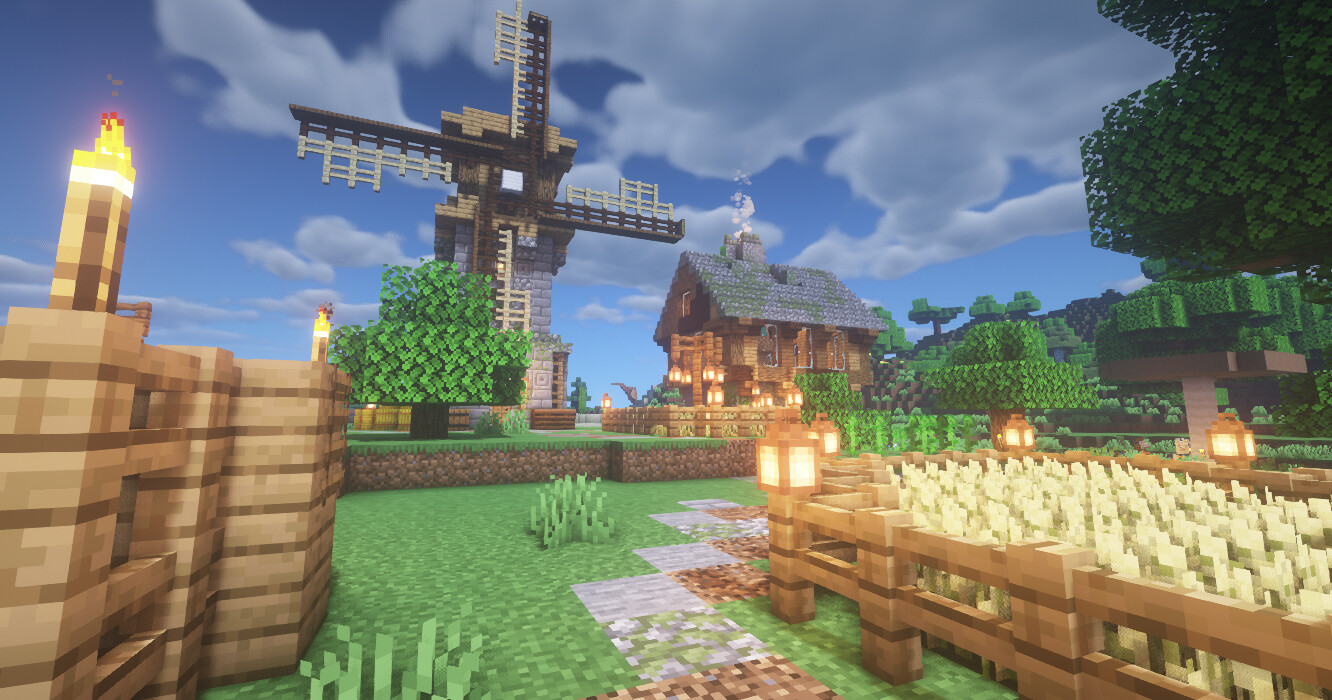This image is a detailed screenshot from the game Minecraft, showcasing an intricately designed in-game environment. Prominently featured in the background is a windmill constructed from what appears to be pixelated fences, with a solid brick base. To the windmill's left, at the base, are lush, square bushes adding a touch of greenery. Towards the right side of the image stands a rustic wooden cabin with a distinctive angled gray roof. Behind the windmill, on the left, there is a fence made of brown, boxy pixelated bricks, which is flanked by two iconic Minecraft torches. These torches are placed symmetrically on both the left and right sides of the fence. The ground in the foreground is carpeted with vibrant pixelated grass. Surrounding a fenced-in crop area is a boxy walkway, providing a clear path around the vegetation. The edges of this cultivated area are adorned with lanterns, illuminating the scene with a warm, pixelated glow.